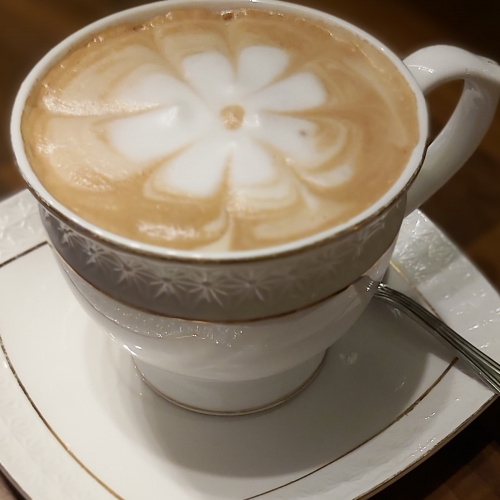This image portrays an elegantly crafted cappuccino served in a delicate white ceramic cup with a matching saucer, both adorned with intricate gold and white sunburst designs. The cappuccino features a beautifully crafted flower pattern made from white milk froth atop the rich brown coffee. The cup, which narrows gracefully towards its base, has a white handle and is almost filled to the brim. Accompanying the cup on the saucer is a silver spoon, positioned such that only its handle is visible, while the rest of it is obscured by the cup. The ensemble rests on a brown wooden table, with the background subtly darkened by the lighting, highlighting the reflective gleam on the cup and saucer.